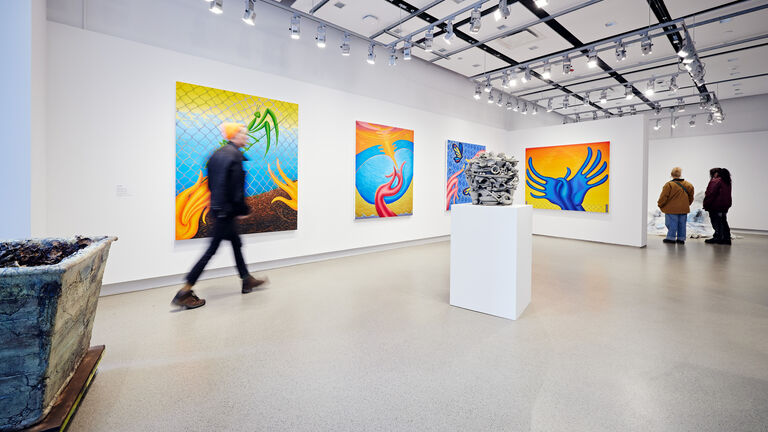The photograph depicts a modern art gallery with pristine white walls and a matching ceiling, intricately outfitted with black scaffolding and silver framing to support several strategically placed silver spotlights. These spotlights are all illuminated, showcasing a series of stylized paintings that adorn the walls and a central artwork. The room's flooring is smooth and gray in color, adding to the contemporary ambiance.

In the center of the room is a white rectangular pedestal, prominently displaying a striking sculpture composed of what appears to be various bones stacked into a cylindrical shape. The paintings on the walls exhibit a variety of vibrant colors including orange, yellow, blue, pink, green, and black. The leftmost painting features a stylized image of a praying mantis.

Additional elements in the scene include another art object situated in the lower left corner, and three visitors to the gallery—one individual walking near the left side and two others positioned towards the top right. The overall setting is that of a museum, marked by its carefully curated artworks and dynamic lighting, attracting the attention and admiration of its visitors.